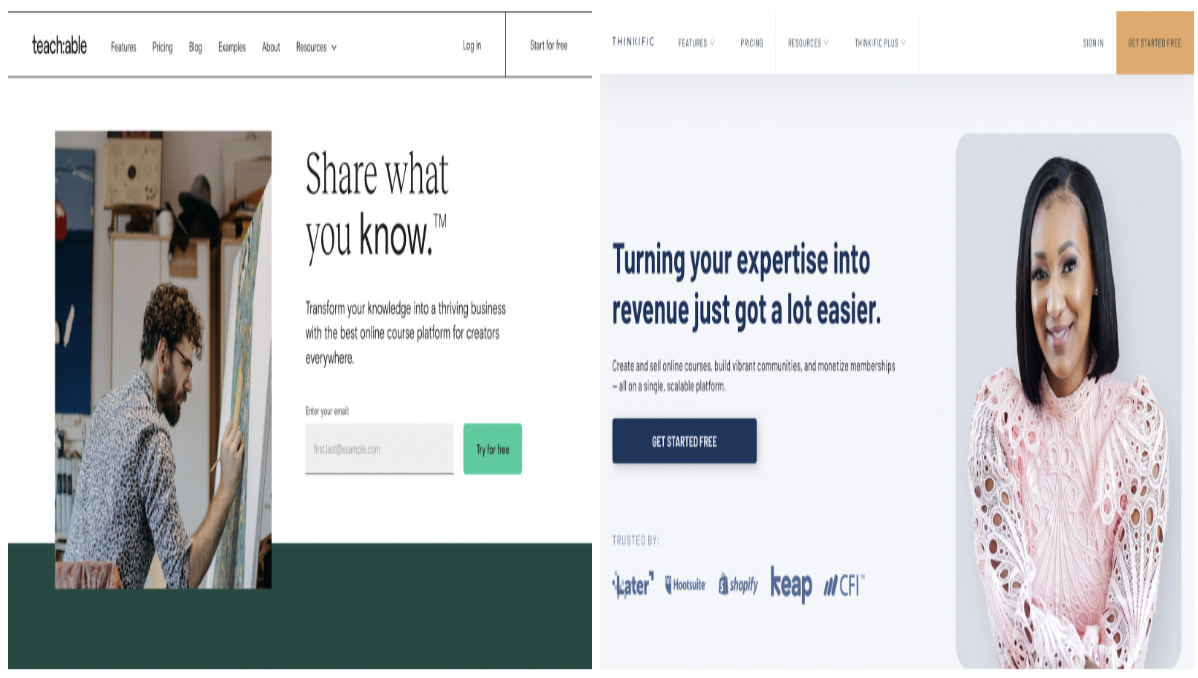The image is a screenshot displaying two webpages side by side, though the quality is noticeably poor with both images appearing compressed and distorted. 

**Left Webpage Description:**
- **Background:** White.
- **Platform:** Teachable (an online platform enabling users to share courses for a fee).
- **Logo:** 'Teachable' in lowercase letters.
- **Menu Options:** Features, Pricing, Blog, Enterprise, About, and possibly Resources.
- **Top Right Corner:** Options for 'Login' and 'Start for Free'.
- **Main Content:** 
  - **Slogan:** “Share What You Know” (with a small TM indicating it's a trademark).
  - **Supporting Text:** "Transform Your Knowledge into a Thriving Business with the Best Online Course Platform for Creators Everywhere."
  - **Email Input:** Gray box for entering an email address.
  - **Call to Action:** Green rounded-corner square with "Try for Free" in dark font.
  - **Photo:** Distorted image of a white man with brown hair and a beard, engaged in drawing (subject of the drawing is unclear).

**Right Webpage Description:**
- **Background:** White at the top transitioning to very light blue below.
- **Platform:** Possibly 'Think Terrific' (exact text unclear due to distortion).
- **Menu Options:** Features, Prices, followed by two unreadable items.
- **Main Content:** 
  - **Slogan:** "Turning Your Experience into Revenue Just Got Easier."
  - **Supporting Text:** (Partially obscured, beginning with "Create").
  - **Photo:** Distorted image of a black woman with medium brown skin, black hair just below chin length, and wearing a pink lace blouse.

There are clear visual signs of compression in both images, making text and elements difficult to interpret precisely.